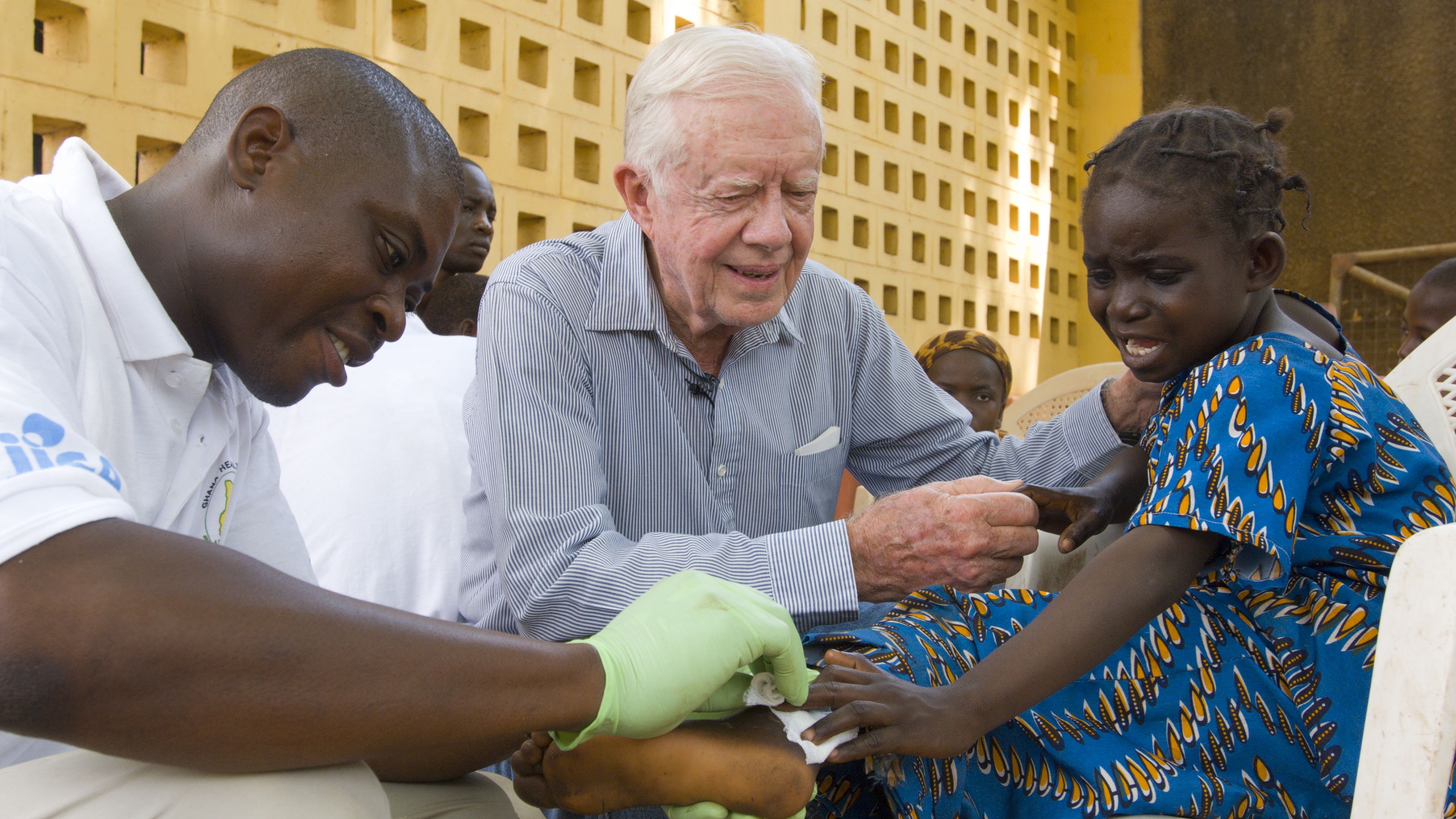In the foreground of this photograph, a young African American girl with braided hair and wearing a blue dress with yellow patterns is seen grimacing as she receives a finger stick to check her blood sugar. Seated on a chair, she appears distressed by the medical procedure. To her left, an African American medical professional, clad in a white nurse's uniform and a green latex hat, is administering the finger stick while wearing a yellow glove. Between them, an older white man with gray hair, wearing a blue-striped, long-sleeved dress shirt and a white handkerchief in his pocket, comforts the girl by resting his hand on her shoulder and holding her right hand. He also appears to have a microphone clipped to his shirt. The background features a yellow wall with numerous small square compartments, and several African Americans are visible, possibly waiting for their turn to be tested.